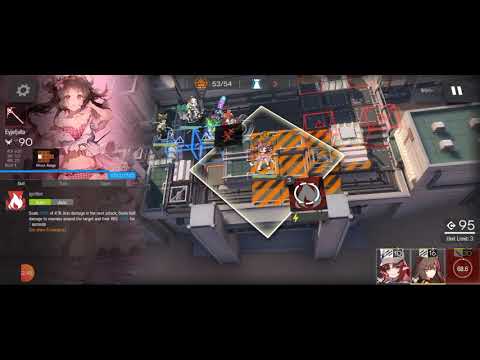The image is a detailed scene from a top-down video game set in what appears to be a robotic, industrial environment. The room features various characters standing at different points, though their exact forms are indistinct. In the center of the scene, a large white diamond shape can be seen, transparent enough to reveal a character beneath it, standing on an orange and gray striped platform supported by gray pillars. To the right, there's another platform topped with a green roof and a building next to it.

In the top left corner of the image, an anime girl is prominently displayed. She is dressed in a skimpy, frilly pink outfit reminiscent of a bathing suit with ruffles. Her brunette hair flows around her, kept back with a flowered band. Beside her are icons: one of a pickaxe and another of a flame. The floor features caution markings in orange, contributing to the industrial, factory-like atmosphere of the game. There are five characters visible in the scene, creating a complex and engaging setting.